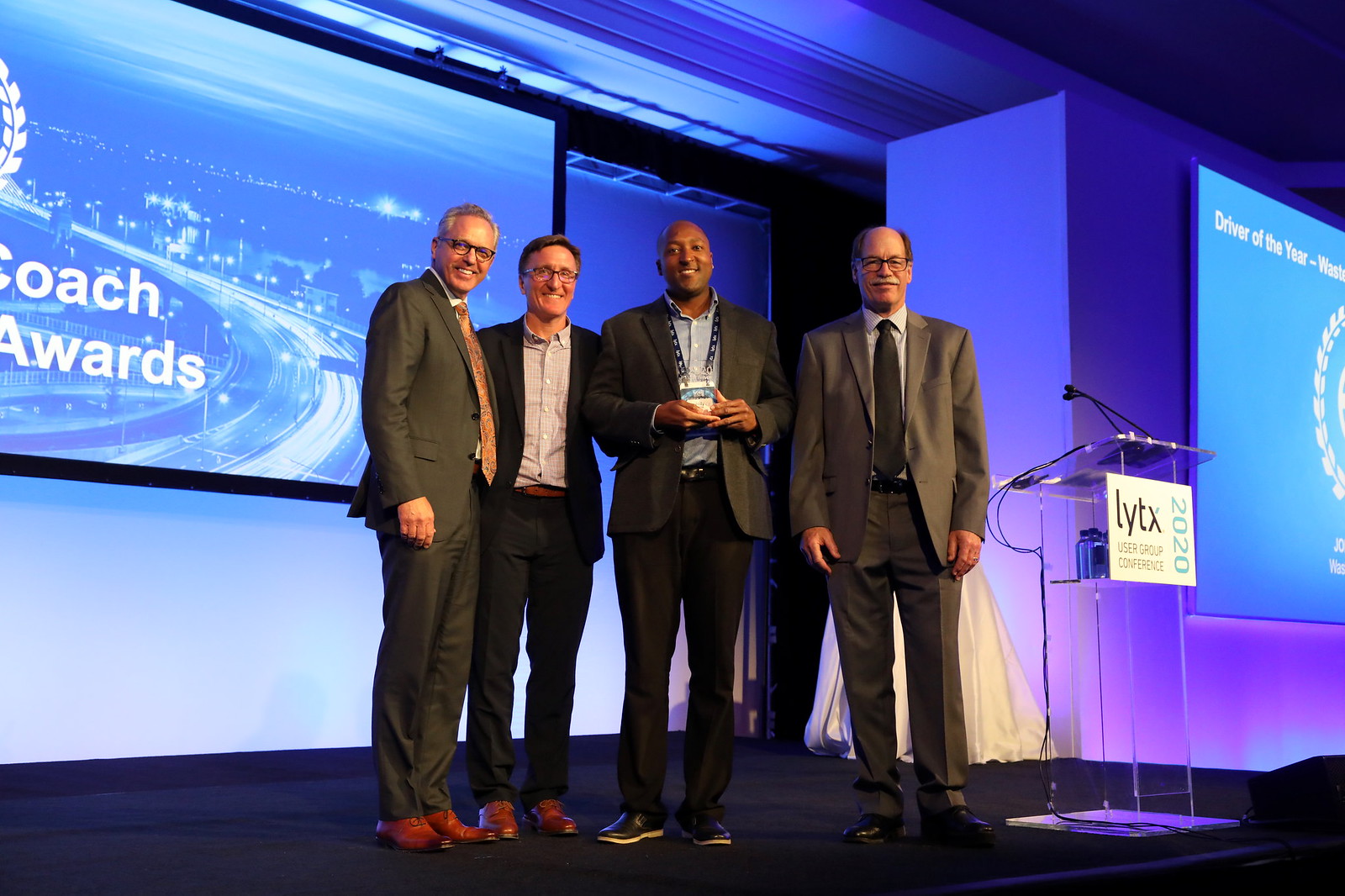In the image, four men are standing side by side on a black stage, under a bluish and purplish-lit background adorned with screens displaying various awards and images. To the right of the men is a clear acrylic podium with a white sign that reads "LYTX 2020" in blue and black text, and a microphone attached to it. 

The man on the far left is wearing a gray suit, brown shoes, glasses, and has partly gray hair. His right arm is down to his side. Next to him stands a man in a black suit with brown shoes, a light blue dress shirt under his jacket, and glasses. 

The third man wears a gray suit with a light blue shirt, a blue lanyard around his neck that holds a white card with a blue stripe and logo, and he has gray shoes. 

The man on the far right is wearing a light gray suit, a slightly darker gray tie, and a light gray or white dress shirt, and he is bald with glasses.

Screens in the background display the words "Driver of the Year" and "Coach Awards" in white text with blue backgrounds showing street and city images. The scene depicts these four individuals on stage, likely for an awards or recognition event.